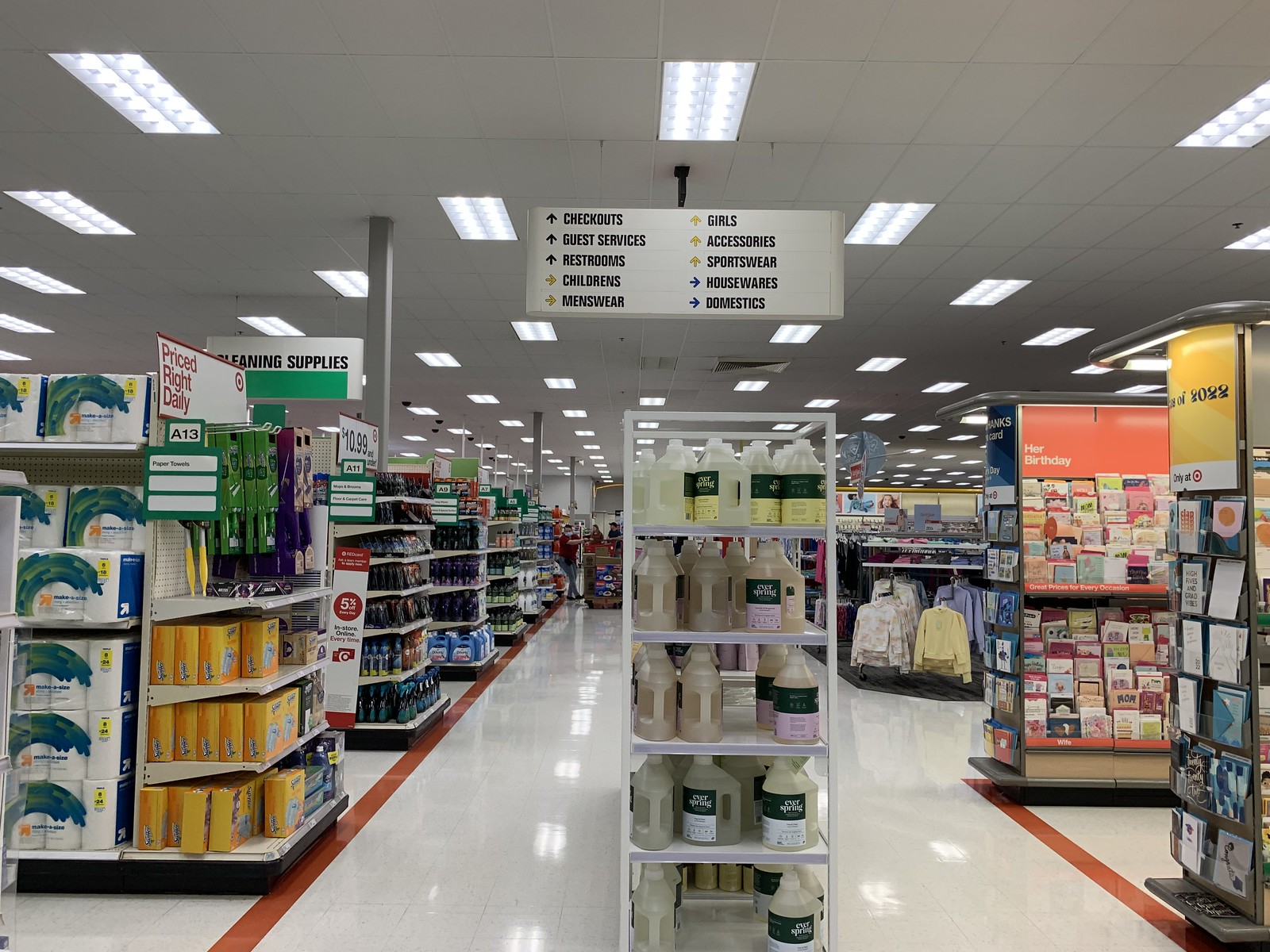In this image of a Target store aisle, we can immediately identify the location by the distinctive red and white signage. To the left-hand corner, a prominent sign reads "Priced Right Daily," accompanied by the familiar Target logo at the top right corner of the sign. Hanging in the top center of the image is a large directional sign that guides shoppers to various departments: Checkout, Guest Services, Restroom, Children's, Men's Wear, Girls', Accessories, Sportswear, Housewares, and Domestics. 

On the right side of the aisle, there is a section filled with greeting cards and stationery. Contrasting this, the left side features shelves stocked with paper towels and cleaning supplies. Dominating the center are Everspring cleaning products, neatly displayed for customers. Further down the aisle, children's clothing is visible, specifically focusing on girls' shirts, showcasing the variety of products offered in this area of the store.